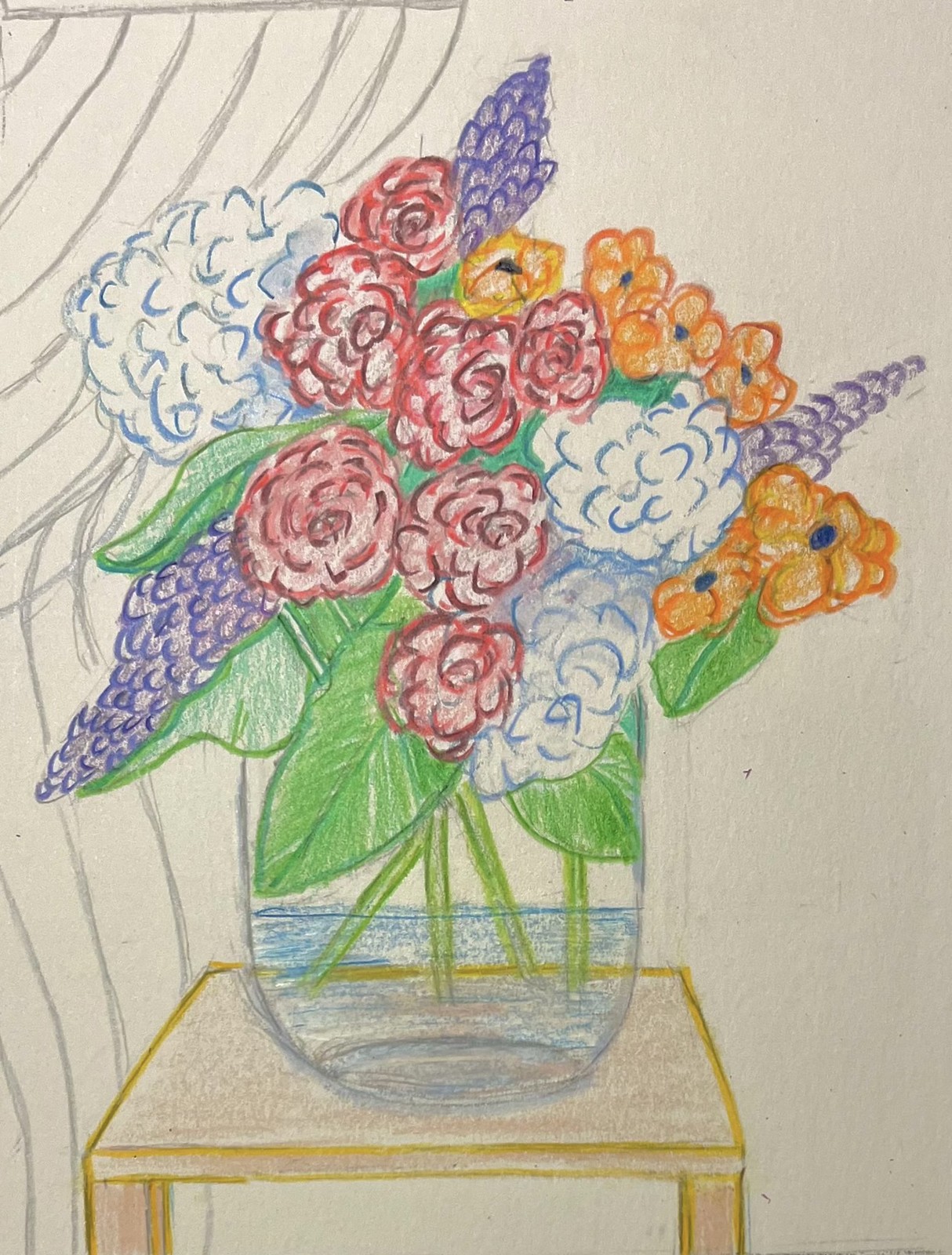This color photograph displays a meticulously detailed line drawing on paper that has a light greyish hue, possibly affected by the lighting conditions. The artwork features an elegant vase brimming with various flowers, most of which are vividly colored. The floral arrangement includes predominantly round pink and orange flowers, the latter adorned with small black dots at their centers, as well as conical-shaped purple flowers. Each bloom is accompanied by large green leaves, adding to the lush appearance. Visible through the round glass vase are the green stems of the flowers, with the vase itself depicted as being half-filled with blue-tinted water. The vase rests upon a brownish wooden stool or table, suggesting a warm, homely setting. To the left side of the image, wavy lines represent a curtain drawn back, adding a dynamic and almost narrative element to the composition.